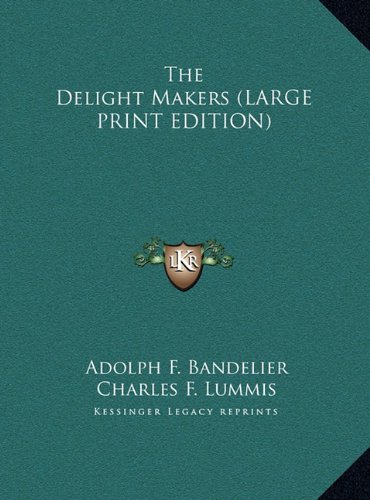The image appears to be the cover of a book with a predominantly jade green textured background. The top and bottom right-hand corners are marked with small black triangles. At the top center of the cover, white text reads "The Delight Makers" with "Large Print Edition" in parentheses underneath. Midway down the cover, a golden shield with a black outline displays the large letter "K" flanked by smaller "L" and "R" on either side. Green vines extend from either side of the shield. Below this emblem, in white text, are the names "Adolf F. Bandelier" and "Charles F. Lummis," with "Kessinger Legacy Reprints" noted in much smaller letters at the very bottom.